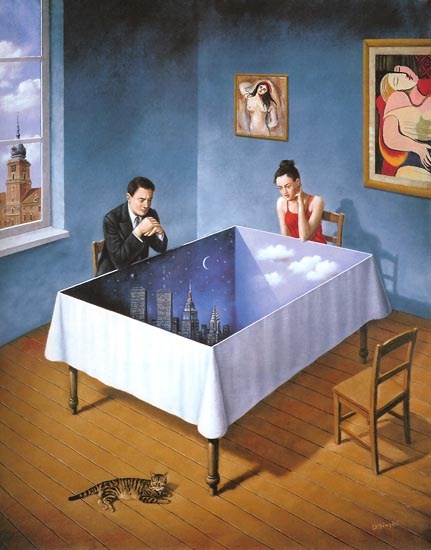In this intricate painting, a man and a woman are seated at a wooden table draped with a white tablecloth, in a room with blue painted walls and wooden floors. The tablecloth features an elaborate depiction of New York City's skyline, blending both night and day elements, with the Twin Towers, the Empire State Building, a smaller building, a moon, stars, and billowy clouds. The woman, dressed in a striking red dress, sits at the head of the table, her left arm bent and her head resting in her hand, giving an air of contemplation. The man in a black suit sits along one side, his elbows on the table and hands clasped, also lost in thought as he gazes at the detailed cityscape. Behind the man is a window showing an ornate building and sky with clouds, while behind the woman, two framed pieces of impressionistic art hang on the wall. An additional wooden chair is placed opposite the man, slightly pushed away from the table. Completing the domestic scene, a striped cat lounges on the floor, adding a touch of warmth to the room.